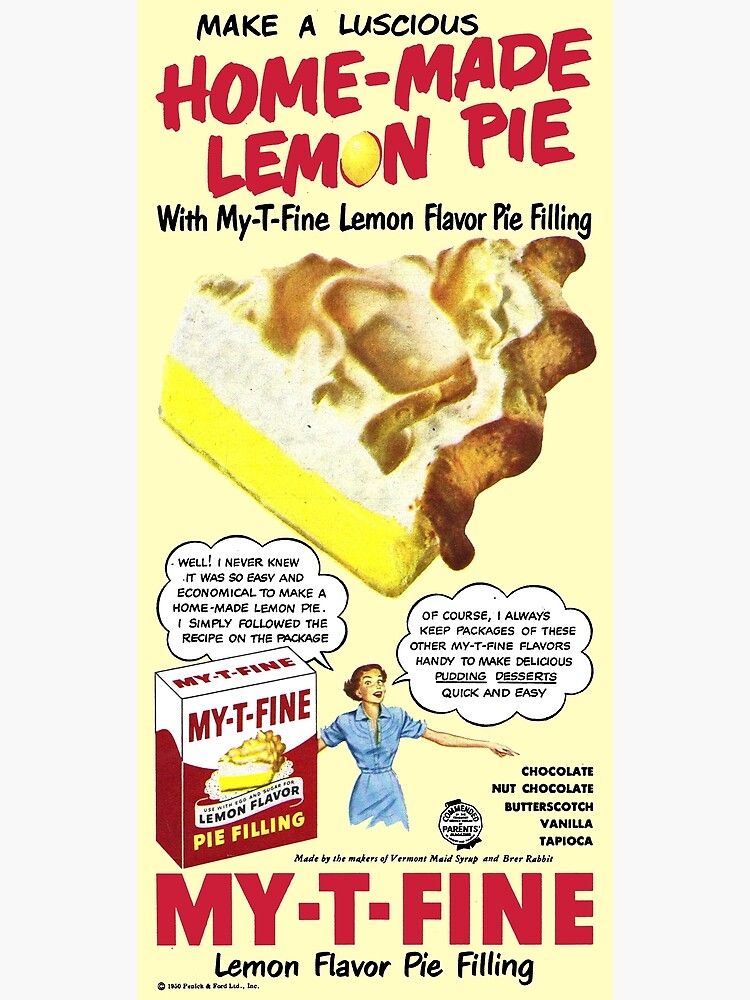The advertisement flyer for Mighty Fine lemon flavor pie filling is a rectangular vintage ad, with the long sides three times the length of the top and bottom sides. It features a large gray border on the left and right, framing a vibrant yellow banner filled with black and red text. Dominating the center is a detailed drawing of a delicious slice of lemon meringue pie, characterized by its golden-brown crust, a bright yellow lemon layer, a white middle layer, and a fluffy meringue topping with a browned peak.

The top of the flyer reads, in bold black text: "Make a Luscious Homemade Lemon Pie." The word "Lemon" is creatively illustrated, with the 'O' shaped like a lemon. Directly below, it continues in black text: "with Mighty Fine Lemon Flavor Pie Filling."

Beneath the visually appealing pie slice is a drawing of a woman in a blue denim dress. She is flanked by two speech bubbles. The left bubble excitedly exclaims, "Well, I never knew it was so easy and economical to make a homemade lemon pie. I simply followed the recipe on the package." Beside her, on the left, is an illustration of the Mighty Fine lemon flavor pie filling box, matching the pie depicted in the center.

The woman's right speech bubble adds, "Of course, I always keep packages of these other Mighty Fine flavors handy to make delicious pudding desserts quick and easy," highlighting additional flavors including chocolate, nut chocolate, butterscotch, vanilla, and tapioca. The bottom of the ad concludes with the brand's name "Mighty Fine" in bold red text, followed by "lemon flavor pie filling."